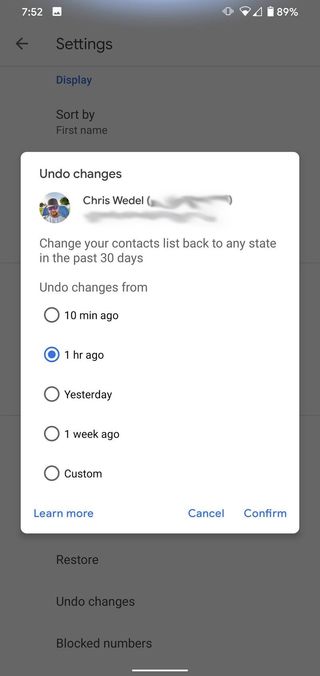The image depicts a smartphone application interface displayed within a small rectangle on a computer screen, simulating a mobile pop-up. The interface is predominantly light gray, punctuated by a large white square in the center. At the top of the gray section, bold black text reads "Sort by" followed by "First Name".

Below this, in the gray section, there are three options listed: "Restore," "Undo Changes," and "Blocked Numbers," suggesting actions users can take to manage changes. 

Within the central white square, more detailed options and information are found. Here, a profile picture of a person named "Chris Weddle" is prominently displayed, showing a bearded individual wearing glasses, a baseball cap, and a white shirt against a backdrop of a sky and field. 

Accompanying this image, the text explains how users can "Change your contact list back to any state in the past 30 days," with options such as "Two changes from 10 minutes ago," "One hour ago" (marked with a blue dot if selected), "Yesterday," "One week ago," and "Custom."

At the bottom of this interface, in a blue font, are three clickable options: "Learn More," "Cancel," and "Confirm."